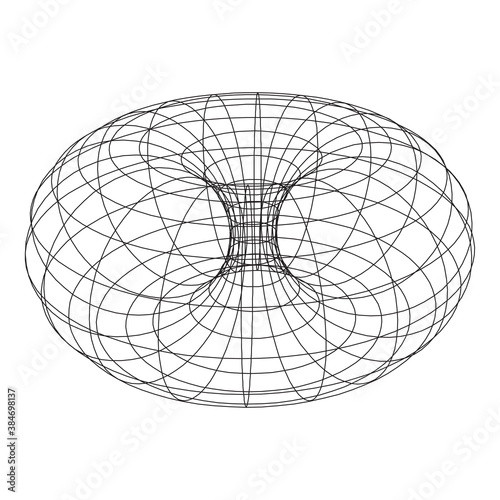The image features a complex structure resembling a hollow spherical shape, meticulously crafted from thin, dark gray or black lines. These lines form an intricate web of symmetrical curvy branches that spirally and radially intersect, creating a visually dense and mesmerizing pattern. The branches are layered horizontally in at least 10 levels, adding depth and dimension to the sphere.

The core of this spherical structure houses an hourglass-like formation composed of two cone shapes; one cone is inverted at the top while the other stands upright at the bottom, converging at their tips. This central design element enhances the focal point and adds a dynamic contrast to the outer branches.

The entire structure sits against a white background, which prominently features Adobe Stock watermarks scattered throughout the image. Additionally, in the lower left-hand corner, there is vertical text displaying "Adobe Stock" followed by a slash and the number 384-698137, acting as a digital watermark for the stock image. The result is a visually striking and detailed illustration with a harmonious blend of geometry and symmetry.